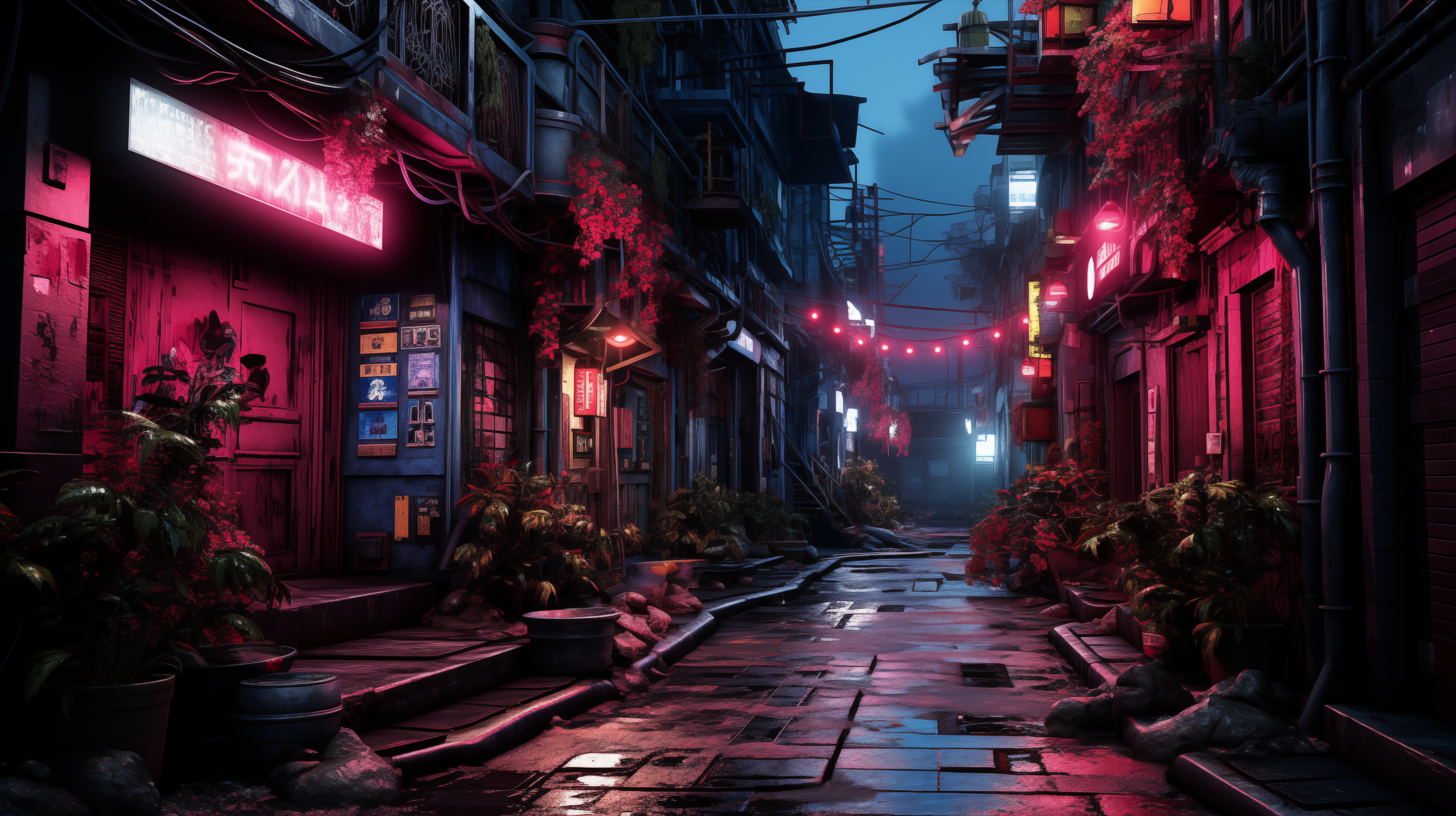This image depicts a vibrant, nighttime scene of an AI-generated oriental city alley. The narrow street, paved with uneven, square cobblestones, glistens as if wet, reflecting the saturated neon lights. Pink and fuchsia neon signs and strings of hanging lights illuminate the area. On the left side, a business with steps leading to red double doors is adorned with a neon sign and various posters on the wall. Further down, another establishment displays its windows and doorway, continuing down the street. On the right side, large water pipes descend the building walls, accompanied by numerous pots of plants and flowers. Though no people are visible, there might be some sitting on the sidewalk. Above the buildings, lantern-like lights add to the bustling yet mysterious urban atmosphere. The far background reveals hints of blue sky, slightly blurred, amidst the predominantly black, dark gray, and deep blue hues.